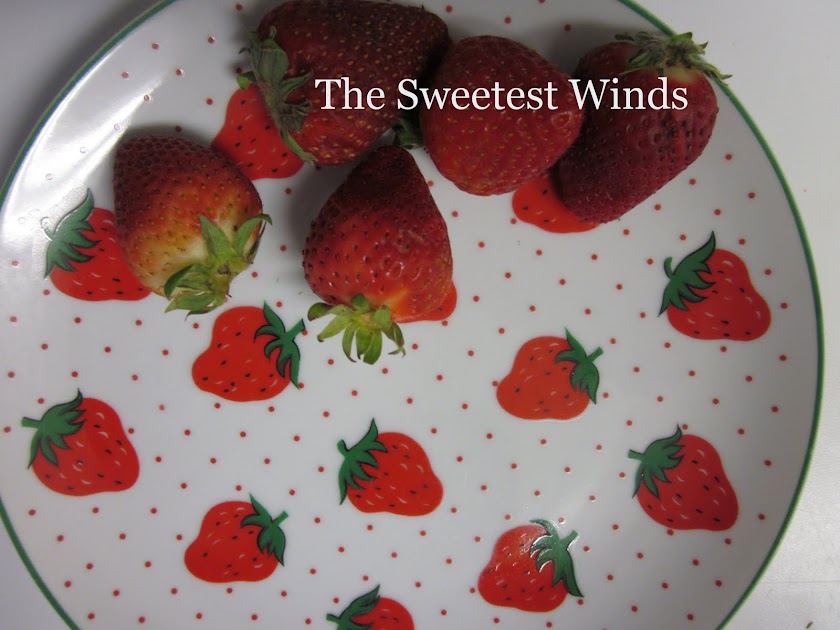The image showcases a predominantly white plate with a thin green border, perfectly complementing the green stems of both the plate’s design and the real strawberries presented. The plate itself is adorned with a pattern of red strawberries and tiny red polka dots arranged in a grid-like formation. Centered towards the top of the plate, there are five real, ripe strawberries with green stems, meticulously arranged in a slight cluster, with three in a line at the top and two positioned below towards the left. On top of these strawberries, white text reads "The Sweetest Wins," lending a playful touch to the presentation. The plate is situated on a white surface, further accentuating its detailed design and the vivid colors of the strawberries, both real and illustrated.